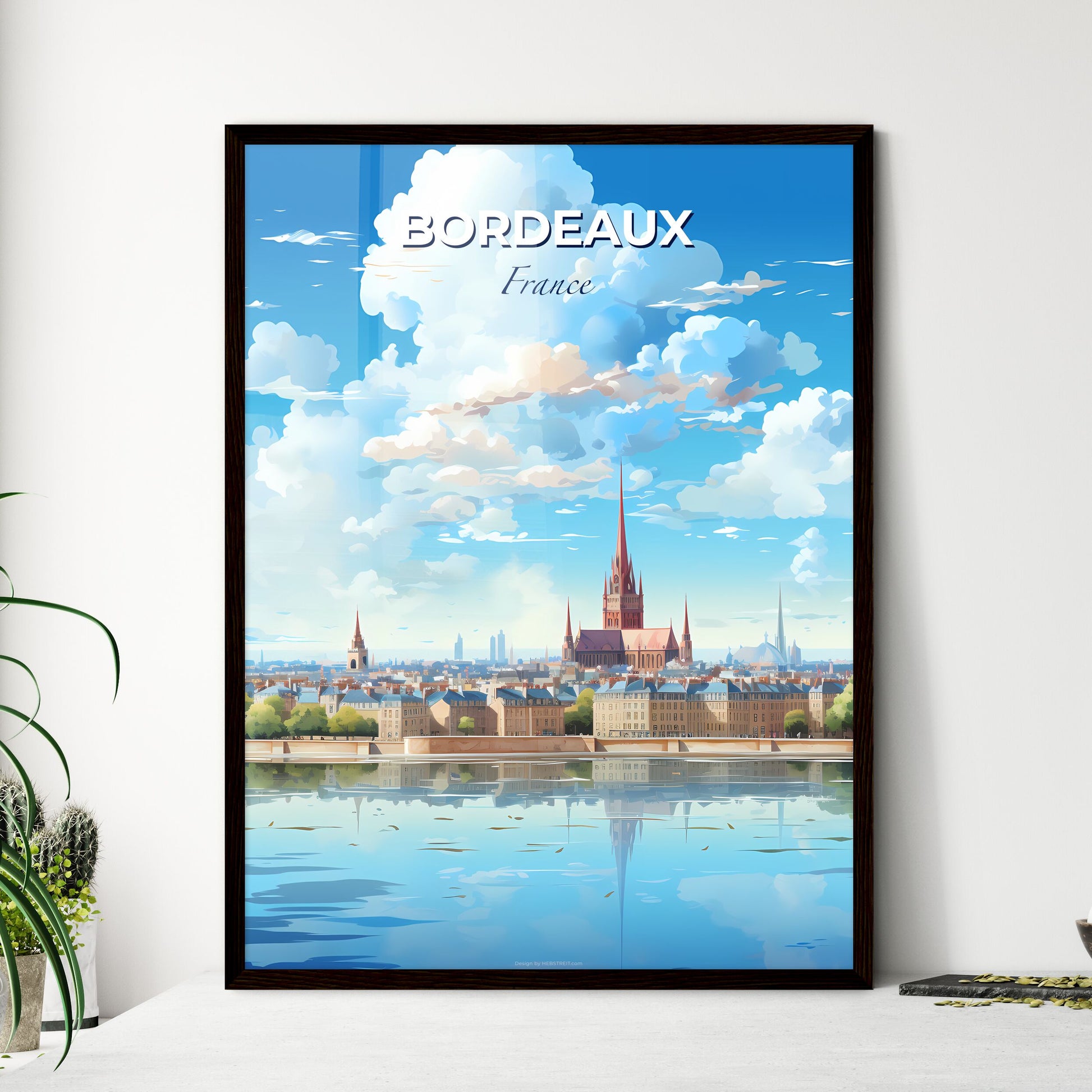This eye-catching poster advertisement for visiting Bordeaux, France is displayed leaning against a white wall, sitting on a pristine white countertop. Framed in a slender black frame, the poster showcases a stunning, computer-generated illustration of the city. At the top, bold white capital letters spell out "BORDEAUX" with "FRANCE" in blue letters beneath it. 

The scene captures the charm of Bordeaux with beautifully depicted blue skies adorned with fluffy white clouds. The cityscape features several tall, pointy-topped buildings, including a prominent church with a high spire reaching toward the sky. In the foreground, a serene waterway reflects the surrounding architecture, adding a sense of tranquility to the vibrant city life depicted. 

Along the left side of the poster, near the edge, from the center to the bottom, are two planters, one gray and one white, containing small cacti and a plant with long green leaves. Off to the right near the bottom is something indistinct in black and yellow. This detailed and inviting visual has no people, vehicles, or animals rendered, allowing viewers to fully appreciate the architectural and natural beauty of Bordeaux. The palette consists of whites, blues, browns, tans, greens, gray, and black, perfectly capturing the essence of the city and its picturesque surroundings.